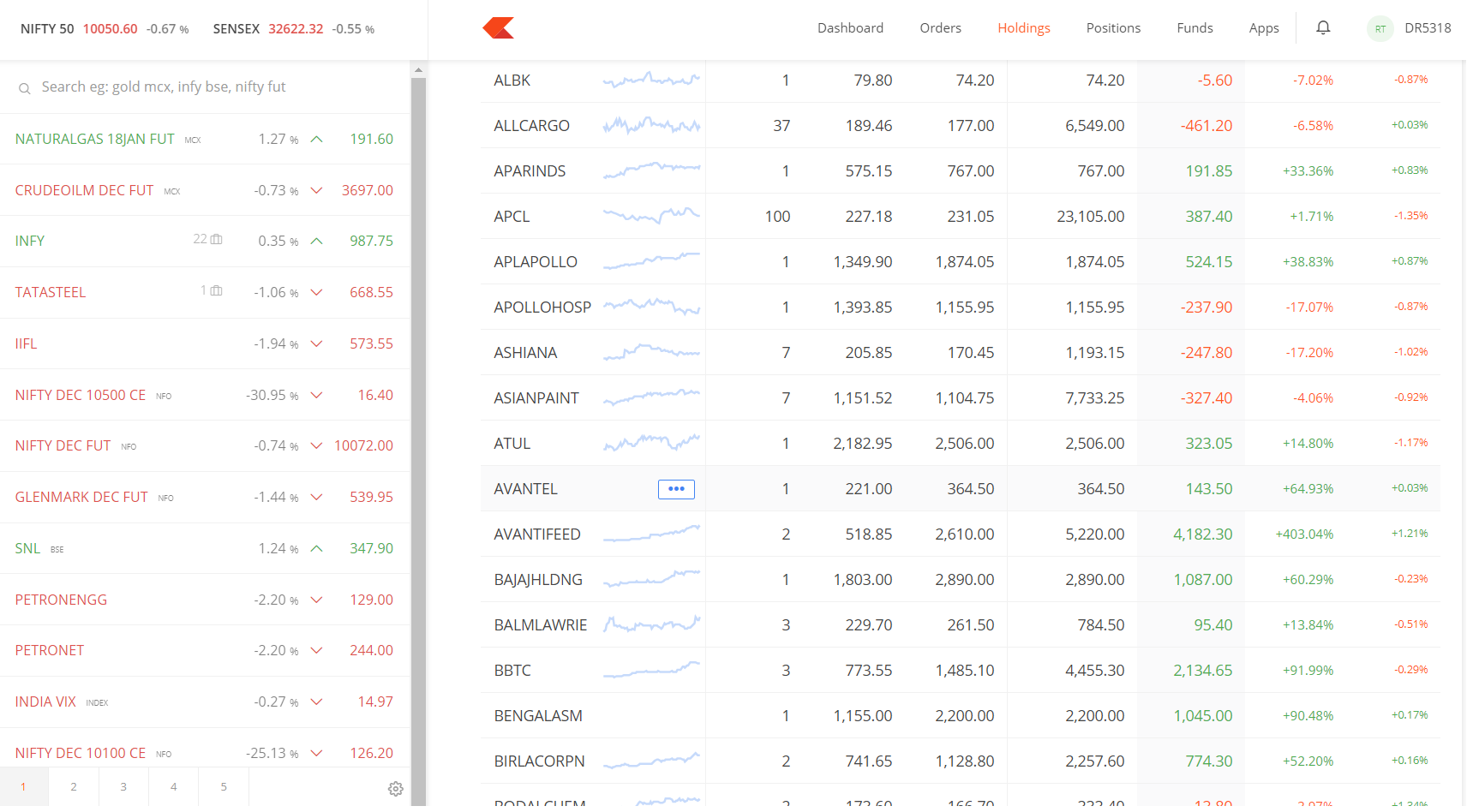The image shows a detailed screenshot of a stock market tracking interface. The background consists of numerous white columns. On the left-hand side, the heading "Nifty 50" is prominently displayed in black, followed by the figure 10,050.60 in red. Below it, the value -0.67% is shown in gray. Further down the screen, another figure 106 is written in black, below which 32,622.32 appears in red, accompanied by -0.55% in gray.

In the top search bar area, it reads "search eg.go, M-C-X, M-C-B-S-E, Nifty F-U-T" in gray. On the right sidebar, labeled in black, are options such as "dashboards" and "borders," while "holdings" is highlighted in red. Black text continues to list "position funds," accompanied by a thin, gray dividing line running vertically down.

Additionally, a gray bell icon with a green circle inside reads "R-T." Just beneath, the code "D-R-5-3-1-8" is displayed in black. A scroll bar on the right-hand side shows a list of stocks with the names: 
- A-L-B-K
- O-R Cargo
- Apparent
- A-P-C-L
- Alpapolo
- Alpapolo
- Asiana
- Asian Paint
- How to
- Avento (highlighted in gray)
- Abitifi
- Bajaj Holden
- Bomb Lawyer
- BBTC
- Bangla Latham
- Bairon Corp

Each stock is listed in succession, creating a comprehensive summary of the available options within the interface.